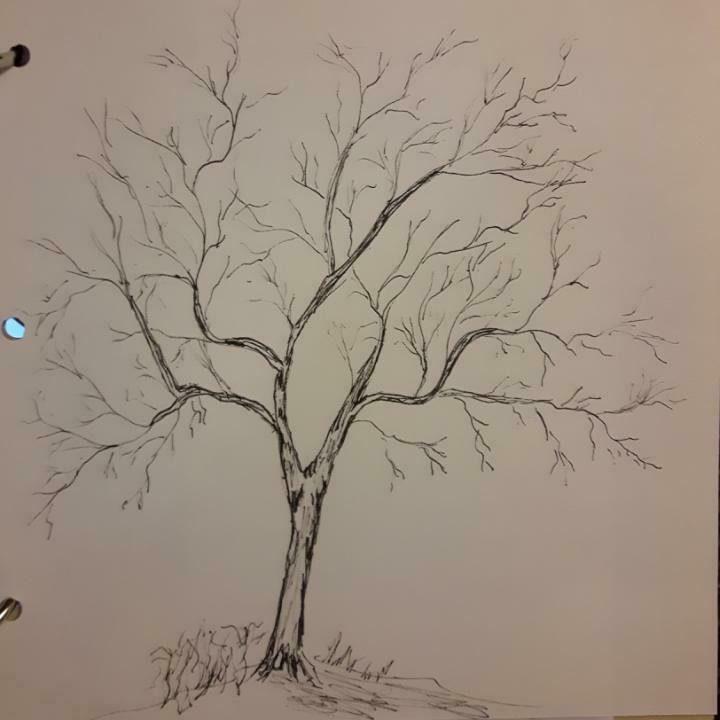The image depicts a simple, yet evocative pencil drawing of a leafless tree on a piece of paper. The paper, which appears to be part of a notebook or held together by metal rings, features three hole punches along the side, two of which are visible. The focal point of the drawing is the tree itself, barren of leaves, suggesting a winter scene. The tree sits atop a gently sloping hill with sparse, sketchy grass beneath it. There is no artist's signature or identification on the drawing. The paper has a unique dark bronze hue, almost leaning towards light burgundy, with slight shading variations that add depth to the background. The lines of the tree are sketchily drawn, lacking intricate detail but clearly delineating the form of a young tree with thin, empty branches. The minimalist style effectively conveys the starkness of winter, despite the absence of snow in the scene.